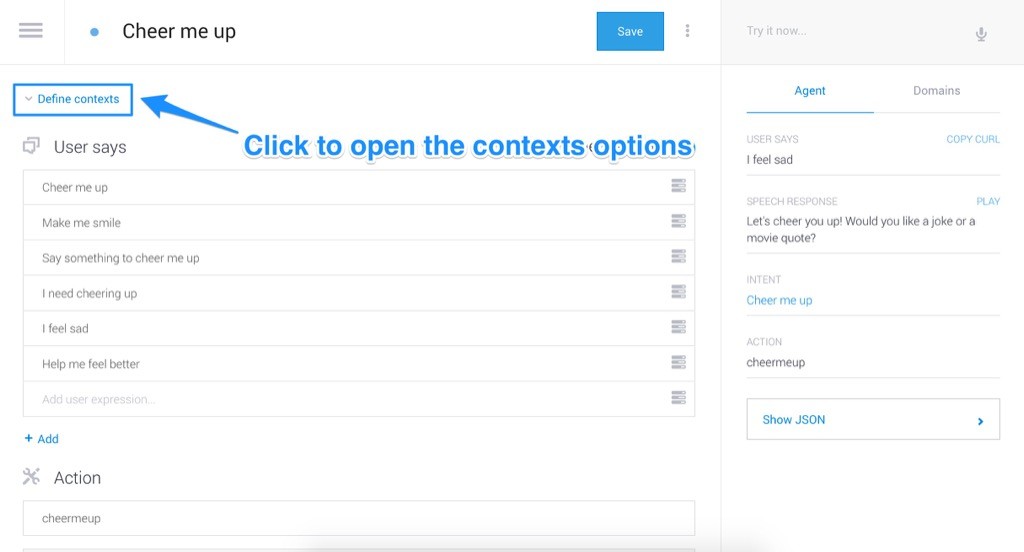The image showcases a detailed user interface (UI) of a chatbot or conversational AI configuration screen, replete with various interactive elements and user inputs. 

At the top left corner, a blue circle is highlighted with the text "Cheer me up." Below it, a blue square with the label "Save" is followed by another element that reads "Try it now" in gray text. Adjacent to this, there is a blue bar with the text "Define context," with an instruction underneath that says, "Click to open the context options."

A central column lists user inputs and possible responses. The column header is "User Says," with examples such as: "Cheer me up," "Make me smile," "Say something to cheer me up," "I need cheering up," "I feel bad," and "Make me feel better." A blue plus sign labeled "It's gear" indicates options for configuring tools and actions under the title "Action: Cheer me up."

On the right, a segmented column displays the text "Try it now" at the top. Beneath it are sections labeled "Agent" (in blue text) and "Domains" (in gray text). One user input example is "I feel sad," which triggers a speech response: "Let's cheer you up. Would you like a joke or a movie recommendation?" The identified intent is "Cheer me up," which prompts the corresponding action. 

At the bottom of this area, there is a gray section labeled "Show JSON," accompanied by a right-facing arrow, indicating additional settings or details. The UI contains multiple square icons or placeholders, each representing different configuration options or steps in the process chain.

This comprehensive layout is likely part of the backend configuration interface for developing and testing chatbot responses and intents, providing various interactive tools and contexts for refining user interactions.